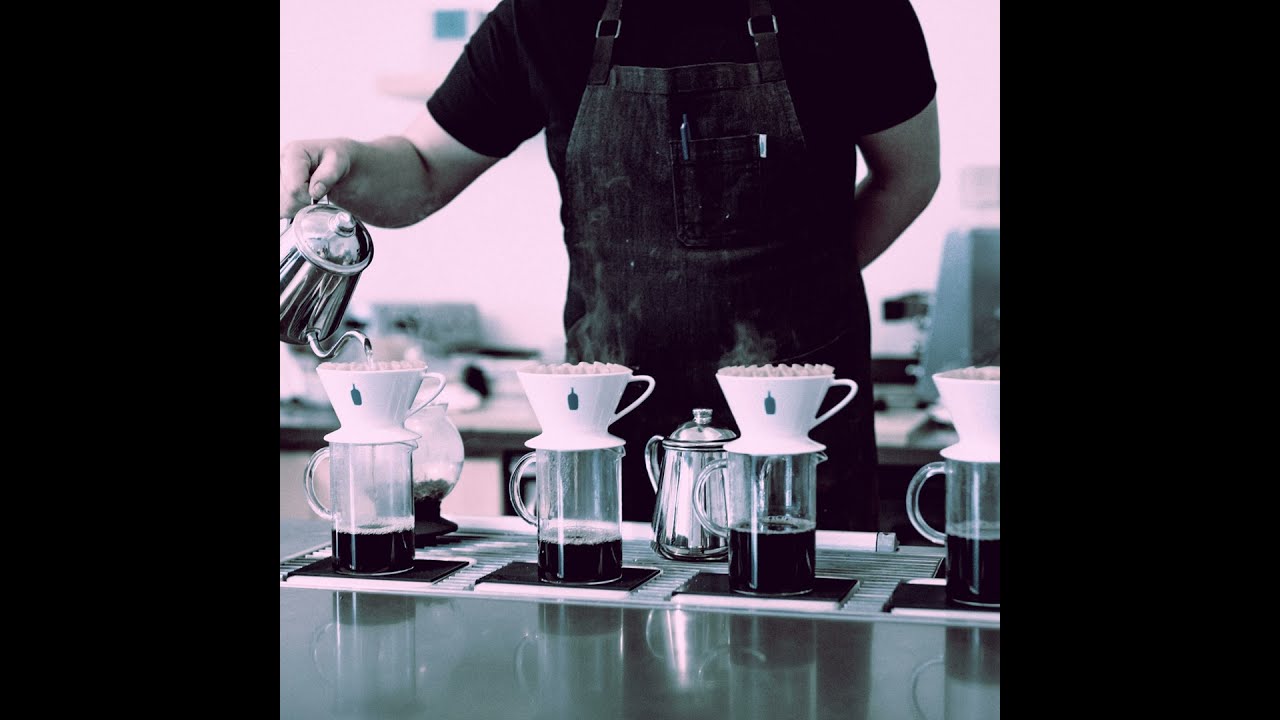The image shows a barista, from the shoulders down, dressed in a black short-sleeved shirt and an apron, poised within a dimly lit coffee shop. The photo is framed by large black borders on the sides. The barista's right hand, extended forward, pours hot water from a silver pot into a white filter set atop a clear glass cup, situated at the far left of four aligned cups. Each clear cup below holds a third of dark liquid, casting reflections on the highly polished surface. A few pins peek out from the apron pocket. To the right, behind the cups, rests another silver pot—possibly for sugar—and a tulip-shaped glass at the left corner. The background reveals a blurry wall and indistinct appliances, further enveloping the scene in a cozy, intimate atmosphere.